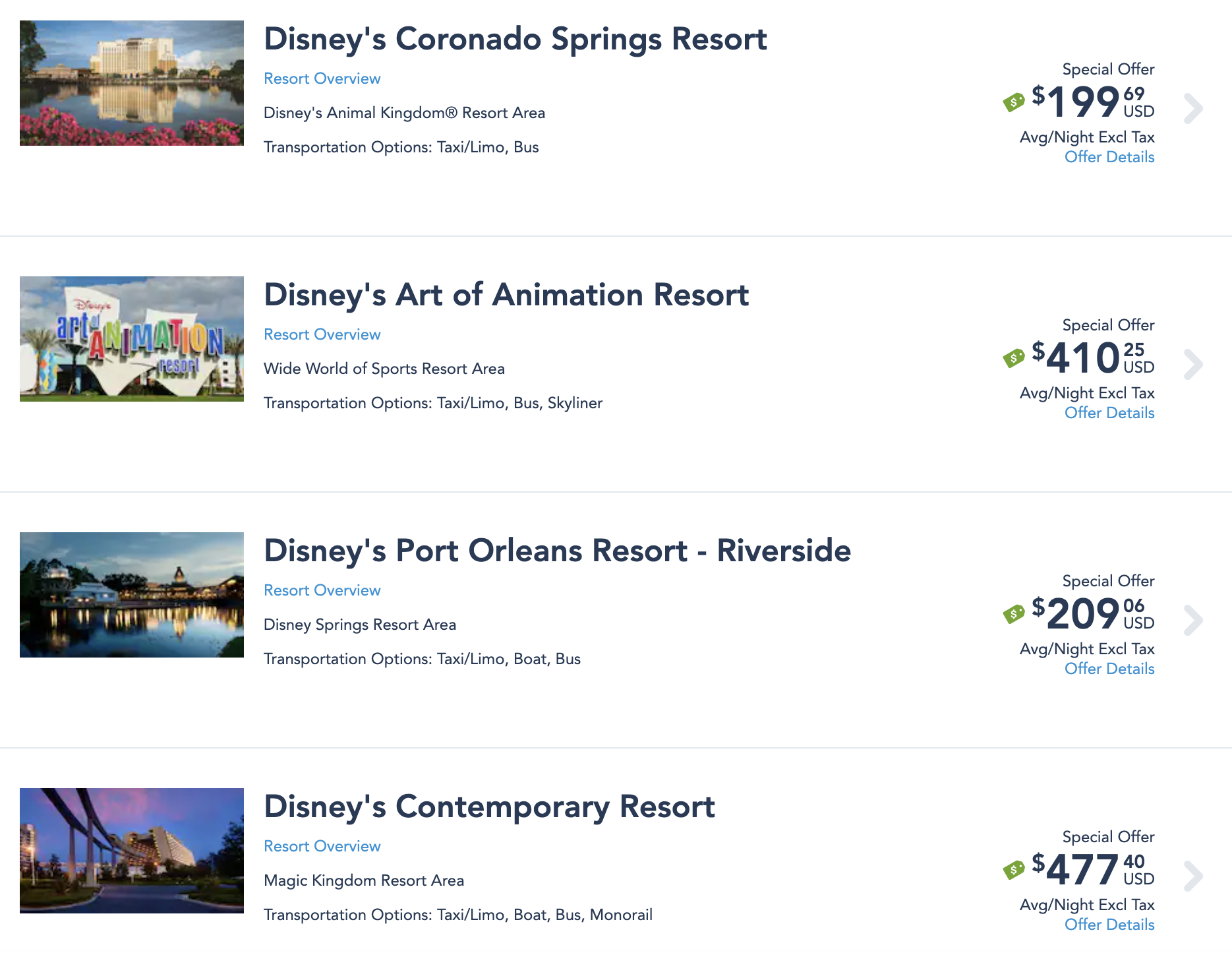On a white background, the Disney website showcases various resort booking options with the following detailed entries:

1. **Disney Colorado Springs Resort**
   - **Location:** Disney's Animal Kingdom Resort Area
   - **Transportation Options:** Taxi, Limo, Bus
   - **Special Offer:** $199.69 USD per night (excluding taxes)
   - **Links:** 
     - "Resort Overview" (in blue)
     - "Offer Deals"
   - **Design:** A light gray line separates this entry from the next

2. **Disney's Art of Animation Resort**
   - **Location:** Wide World of Sports Resort Area
   - **Transportation Options:** Taxi, Limo, Bus, Skyliner
   - **Special Offer:** $410.25 USD per night (excluding taxes)
   - **Links:** 
     - "Resort Overview" (in blue) 
     - "Offer Deals" (in blue)

3. **Disney's Port Orleans Resort - Riverside**
   - **Location:** Disney Springs Resort Area
   - **Transportation Options:** Taxi, Limo, Boat, Bus
   - **Special Offer:** $209.06 USD per night (excluding taxes)
   - **Links:**
     - "Resort Overview" (in blue)
     - "Offer Deals"

Each resort features a photograph on the left side of its description with distinct offers and transportation details.